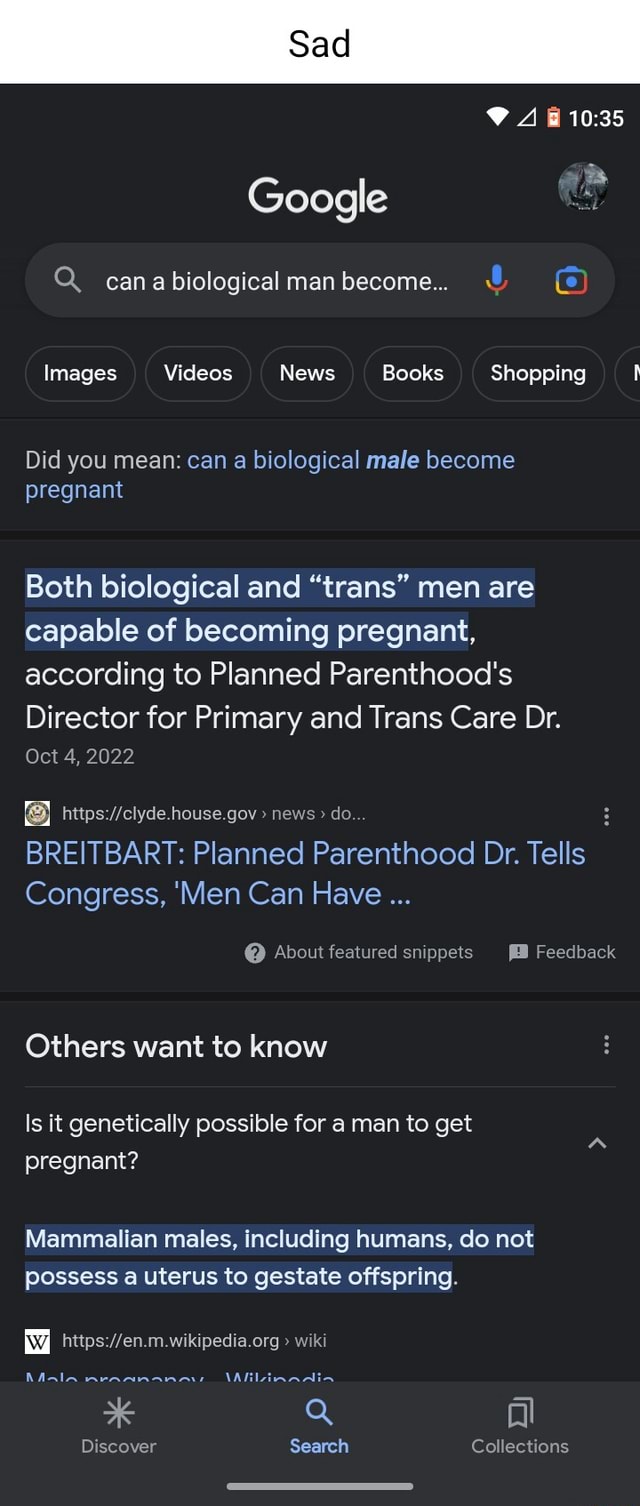The image is a screenshot captured from a mobile device set to night mode, featuring a predominantly black background. At the top of the screenshot, there's the text "SAD" in black letters separate from the phone’s display. 

Within the screenshot, the status bar at the top right shows a full Wi-Fi signal, an empty cellular signal strength, and a battery icon with an orange and white color scheme displaying "10:35" in white digits. Central to the screenshot is the Google search interface with the search box filled with the incomplete query, "can a biological man become...". The search box is a lighter gray with a search icon, and adjacent to this are the blue and red microphone logo and the multicolored (blue, red, and yellow) video or photo logo.

Below the search box, there are category links for different types of searches: images, videos, news, books, and shopping. Underneath this, in gray text, there's a "Did you mean:" suggestion that switches to blue, bolded text with the phrase "can a biological male become pregnant." The main highlighted search result explains, "Both biological and trans men are capable of becoming pregnant," followed by a non-highlighted citation stating, "according to Planned Parenthood's director for primary and trans care doctor."

Following this, there's a snippet from a Breitbart article and an "Others want to know" section showing a related question: "Is it genetically possible for a man to get pregnant?" The highlighted answer states, "Mammalian males, including humans, do not possess a uterus to gestate offspring." Below this, there's a result from Wikipedia.

At the bottom of the screen, the navigation bar features a "Discover" button, a blue "Search" button, and a gray "Collections" button.